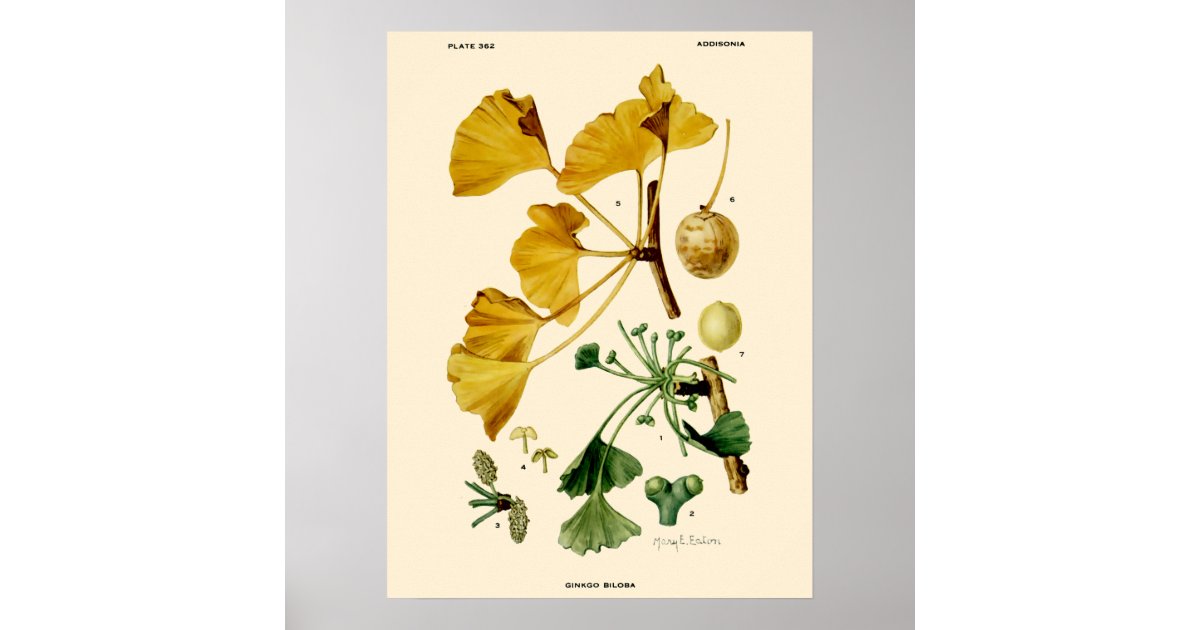This is an intricately detailed botanical plate of the Ginkgo biloba plant, illustrated by Mary E. Eaton. The composition is set against a pale yellow, tan-brownish background, framed within a gray square that transitions from light to dark gray. The upper left corner is marked with "Plate 362" and the right side is inscribed with "Addisonia." 

Central to the plate are various stages of the Ginkgo biloba's growth, meticulously labeled and displayed. The top section features iconic yellow Ginkgo leaves in a half-fan shape, supported by yellow stems that connect to a brown branch. The adjacent right side introduces the seed pod labeled as "number six," alongside the unripened seed pod designated as "number seven." Directly below, green Ginkgo leaves are depicted, transitioning to the right into a detailed illustration of the flowers and stamen.

In the middle of the image, green leaves cascade downward, attached to a stick that appears broken, its fragments showing darker brown, seemingly aged leaves. Below the broken stick, two fruit-like formations are illustrated: a circular nut or fruit with a stem, and beneath it, a smaller cream-colored acorn-like shape without a cap.

Collectively, this botanical illustration exquisitely captures the distinct phases of the Ginkgo biloba plant, presenting its beauty and botanical complexity.